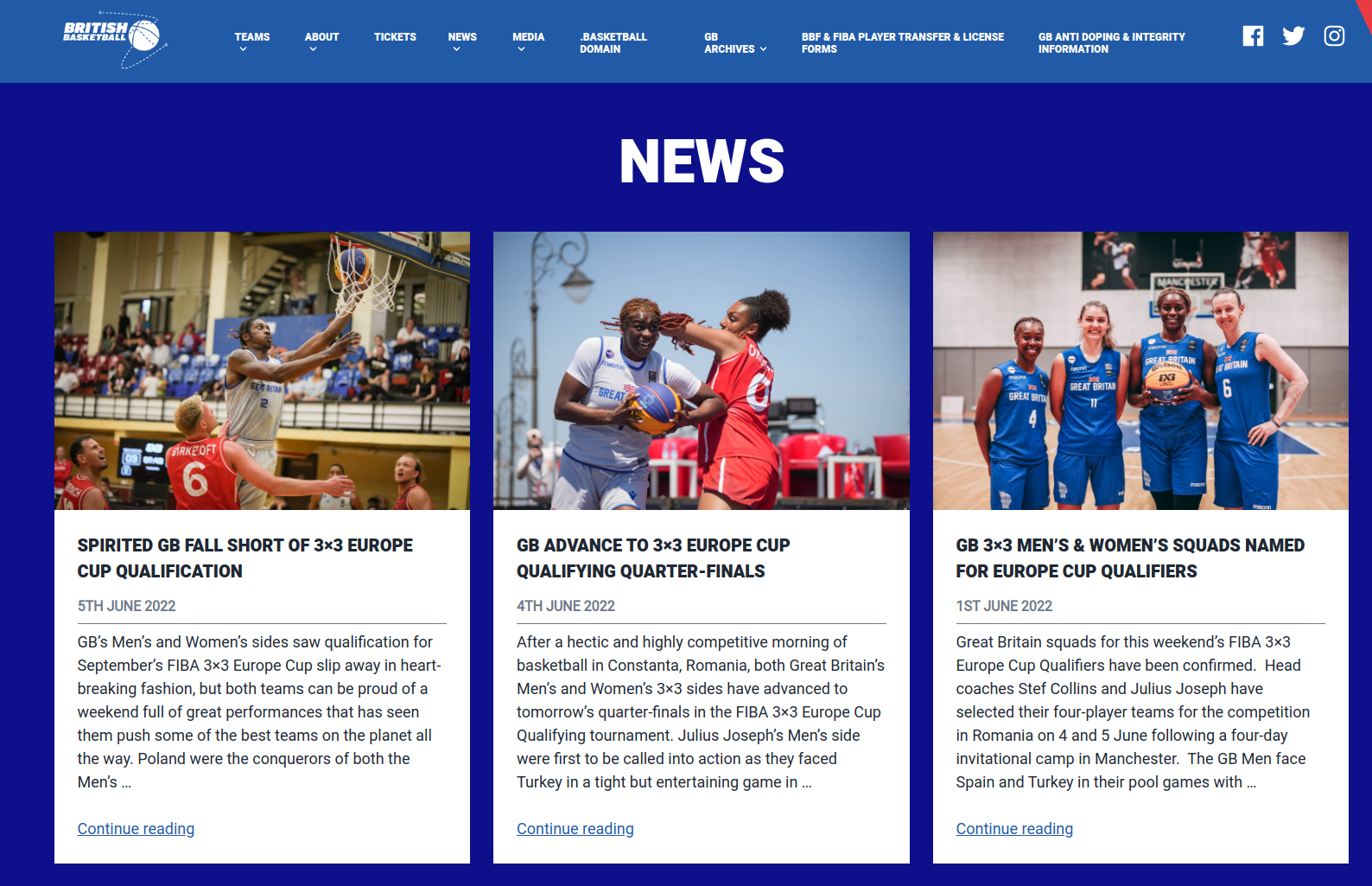This rectangular image, oriented with its longer side horizontally, displays a structured interface with a prominent blue banner at the top featuring white text. The banner reads "British Basketball," accompanied by a basketball icon. Moving right along the banner, there are designated tabs labeled: "Teams," "About," "Tickets," "News," "Media," and "Basketball Domain." Positioned centrally on the page are links to "GB Archives," "Transfer and License Forms," and "GB Anti-Doping and Integrity Information." On the far right of this top section, there are social media icons for Facebook, Twitter, and Instagram.

Below this banner, the background transitions to a dark blue with "News" prominently displayed in white text in the middle. This section is divided into three columns, each showcasing an article with an image, title, and descriptive paragraph. The titles are as follows: 

1. "Spirited GB Falls Short of 3x3 Europe Cup Qualification," dated June 5, 2022, on the left.
2. "GB Advance to 3x3 Europe Cup Qualifying Quarterfinals" in the middle.
3. "GB 3x3 Men's and Women's Squads Named for Europe Cup Qualifiers" on the right.

Each article features an accompanying image and a brief summary paragraph underneath the title.